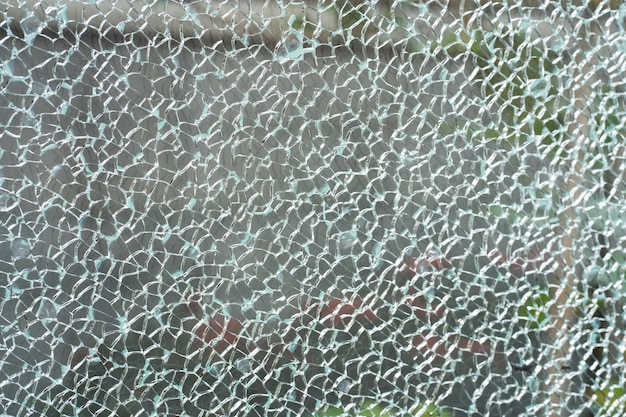This image features a striking display of shattered tempered glass. The fractured glass appears in hundreds of pieces, each roughly an inch in size, creating a mosaic-like pattern. The transparency of the glass has been heavily obscured due to the intricate web of cracks spreading throughout the pane. Although the specific details behind the cracked glass are ambiguous, there are hints of a background scene. At the bottom, there may be five or six goldfish, with four aligned from the center to the right and another positioned below, near the third one on the right. In the upper right area, glimpses of what seem to be green leaves can be discerned, extending down the right edge and intertwined beneath the perceived goldfish at the bottom. Additionally, vague impressions of a tree, possibly with red elements such as a motorcycle, hint at a more complex backdrop. The overall effect of the cracked tempered glass, distorted yet detailed, imparts a visually compelling image that intricately blends texture and color.